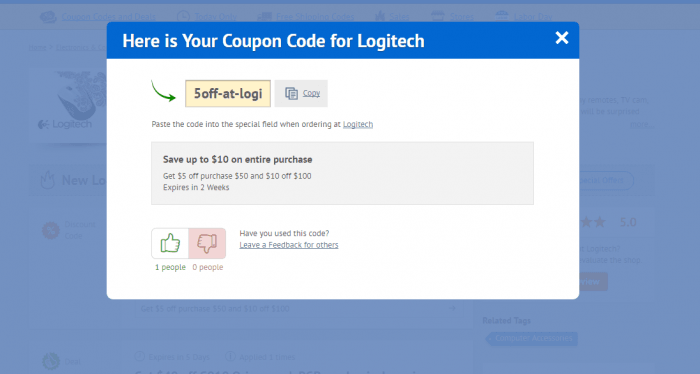The image displays a pop-up menu on the Logitech website. In the blurred background, various elements of the site are visible, including a picture of a mouse, sections showcasing new Logitech products, and other shopping options, complete with star ratings. The backdrop is partially obscured by a translucent light blue overlay, drawing attention to the pop-up panel in the center.

The pop-up panel features a blue bar at the top with text offering a coupon code for Logitech. A close button is situated in the upper right-hand corner. Below the blue bar, there is a white area containing further details. A green arrow swoops down toward a yellow rectangle with a thin gray border, which contains the coupon code "five off - at - Logi". Adjacent to this is a copy icon and blue text on a pink background that instructs users to paste the code in the designated field when ordering.

Further down, a gray rectangle contains promotional details: "Save up to $10 on your entire purchase. Get $5 off on purchases of $50, and $10 off on $100." It also notes that these offers expire in two weeks. At the bottom of the pop-up, there are upvote and downvote buttons for user feedback, with the green upvote marked and the pink downvote unchecked. The panel also asks users to indicate if they have used the code and provides a link for leaving feedback for others.